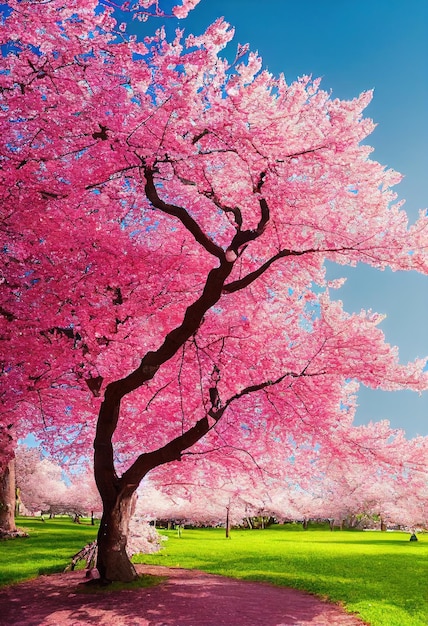This image depicts a vivid and vibrant scene dominated by a Japanese cherry blossom tree in full bloom. The tree stands front and center, showcasing a trunk with dark brown bark and an abundance of bright pink flowers. The blossoms range in hues from light to dark pink and even white, creating a striking contrast against the clear, blue, cloudless sky. The background features a park area with numerous other cherry blossom trees also in bloom, their pale pink and white petals blending harmoniously into the distant landscape. Surrounding the central tree is a meticulously maintained patch of ground, bordered with mulch that forms a clean island of sorts, adding to the orderly feel of the scene. This mulched area appears to have a pinkish hue, possibly from fallen petals. The grass enveloping this area is lush, fresh, and vividly green, contributing to the overall beauty of this sunny, clear day devoid of human or animal presence. The winding branches of the central tree add character to the composition, making this photograph a stunning portrayal of nature’s springtime splendor.